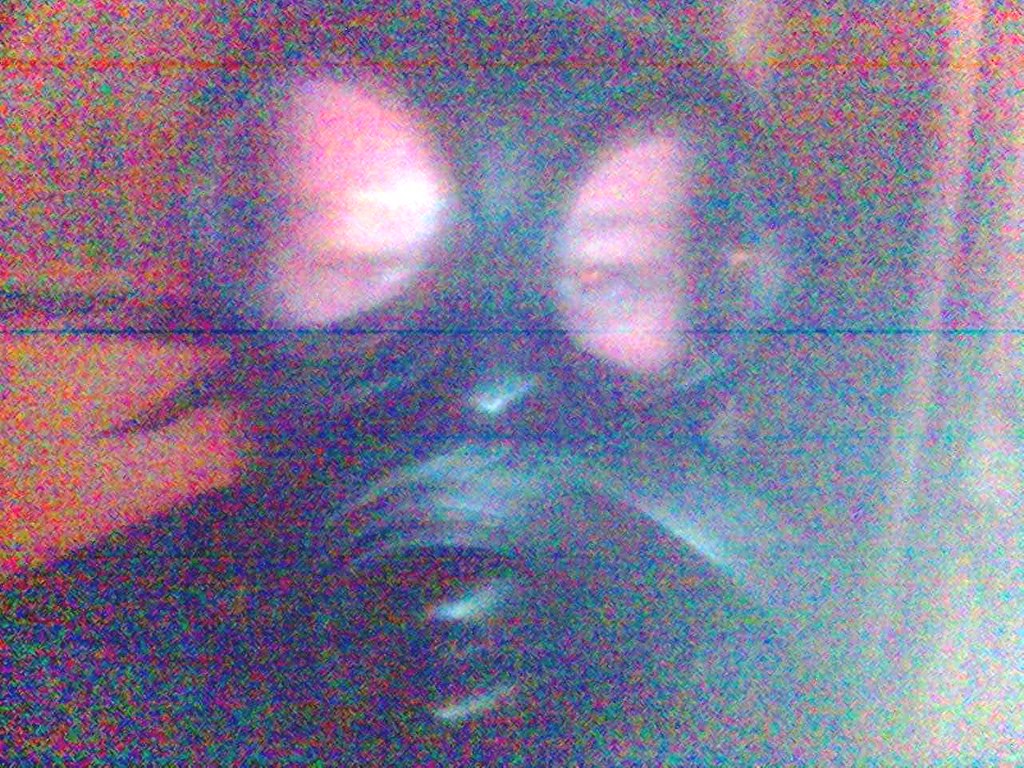In the image, we see a very grainy, rainbow-colored static effect that makes it look as if it was captured by a low-quality webcam or taken off a screen. Despite the static, you can discern a white individual—whose gender is indeterminate—looking directly at the camera. They are wearing a black gas mask, with light pink shading around the eyes, and their eyebrows and some skin around the eyes are visible through the eye holes in the mask. The person is dressed entirely in black, blending into the overall dark appearance of the mask. The background is filled with colorful static, reminiscent of TV static, but rainbow-hued instead of the typical black and white. To the left, there's a faint pink tint, possibly a photo hung on the wall, and to the right, a curtain can just be made out, suggesting that the photo was taken indoors.